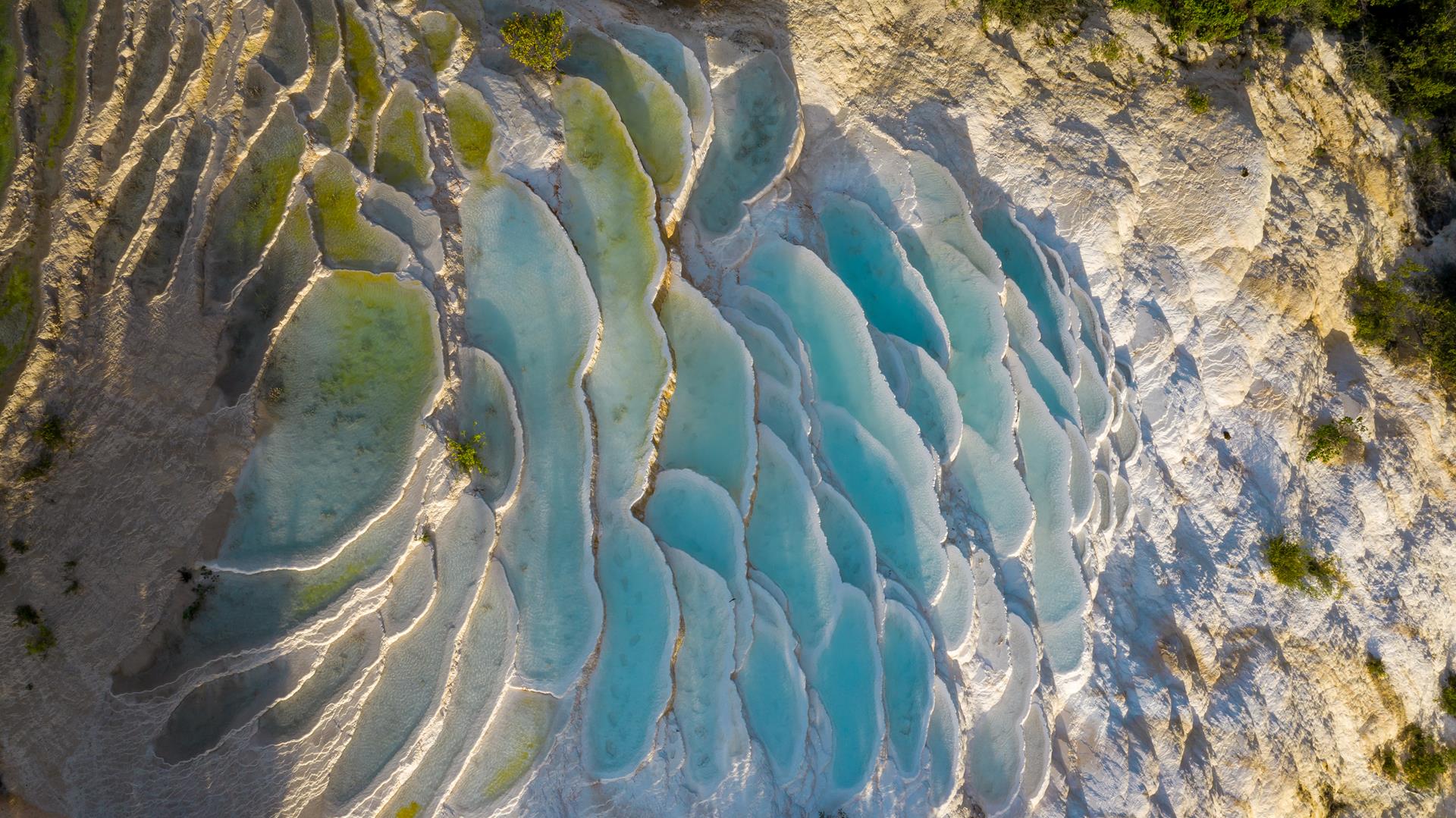The image depicts an aerial view of a series of tiered salt flats cascading down the side of a cliff, reminiscent of fish scales with their flat, flaring edges. Each tier is filled with light blue water, hinting at the presence of algae, particularly noticeable as a greenish hue towards the sunlit top. The uppermost levels exhibit greenery, including trees and bushes, amidst the rocky surface. Shadows from the setting sun cast high contrast across the scene, obscuring some details and accentuating the texture and depth of the landscape. The edges of the platforms are teal blue, giving the impression of water trapped in the rock formations. The background features white rocks that grow darker as they descend, with additional green shrubbery interspersed throughout. The overall effect is both natural and surreal, resembling a work of art.